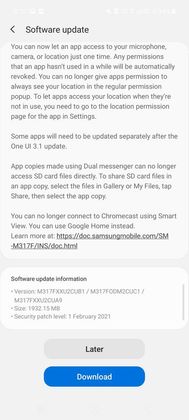**Detailed Caption for Android Software Update Image**

The image displayed on an Android phone screens focuses on a detailed software update notification. At the top, the headline reads "Software Update" with a return caret icon located to its left.

The main body of the text outlines several key changes and improvements:

1. **Permission Updates**:
   - Users can now grant apps access to their microphone, carriers, or location on a one-time basis only.
   - Any permissions not used by an app in a while will be automatically revoked.
   - Users can no longer grant apps continuous location access through the regular permission pop-up. Instead, granting this access requires navigating to the location permission page for the specific app in the settings menu.

2. **App-Specific Updates**:
   - Some apps may require separate updates following the installation of the One UI 3.1 update, which is Samsung's custom skin layered on top of Android.

3. **Dual Messenger Restrictions**:
   - Copies of apps made using the Dual Messenger feature are now restricted from directly accessing SD card files. To share SD card files within these app copies, users must select the files in either the Gallery or My Files app, tap on the share option, and then choose the appropriate app copy.

4. **Chromecast and Smart View Compatibility**:
   - Smart View no longer supports direct connectivity to Chromecast. Instead, users are advised to use Google Home for this functionality. More information can be accessed via a provided URL.

Below this informative section, a box titled "Software Update Information" provides additional details:
- **Version**: Specifies a lengthy version string.
- **Size**: 1932 megabytes
- **Security Patch Level**: 1 February 2021

At the bottom, there are two buttons available for user action: "Download" and "Later".